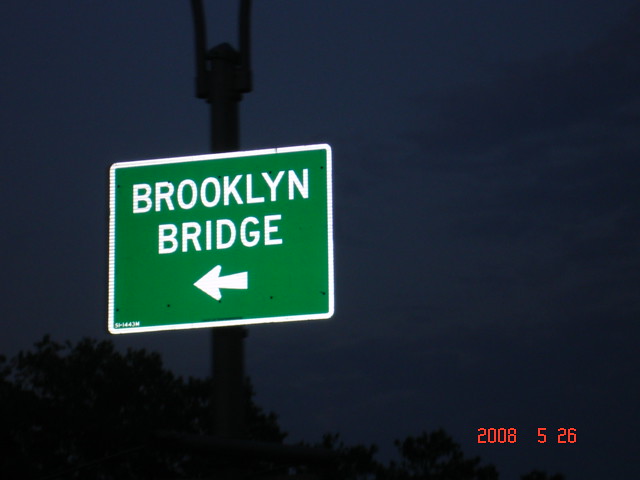A night-time photograph captures a highway sign bathed in illumination against a dark backdrop. The green sign, bordered with white trim, reads 'Brooklyn Bridge' and features a left-pointing arrow, directing drivers towards the iconic landmark. The sign is mounted on a barely visible post, its silhouette faintly discernible in the dim light. Adding to the scene's dated ambiance, an orange-red timestamp at the bottom of the image indicates '2008 526.' In the lower left corner, the shadowy outline of bushes or shrubs subtly enters the frame, adding texture to the composition.